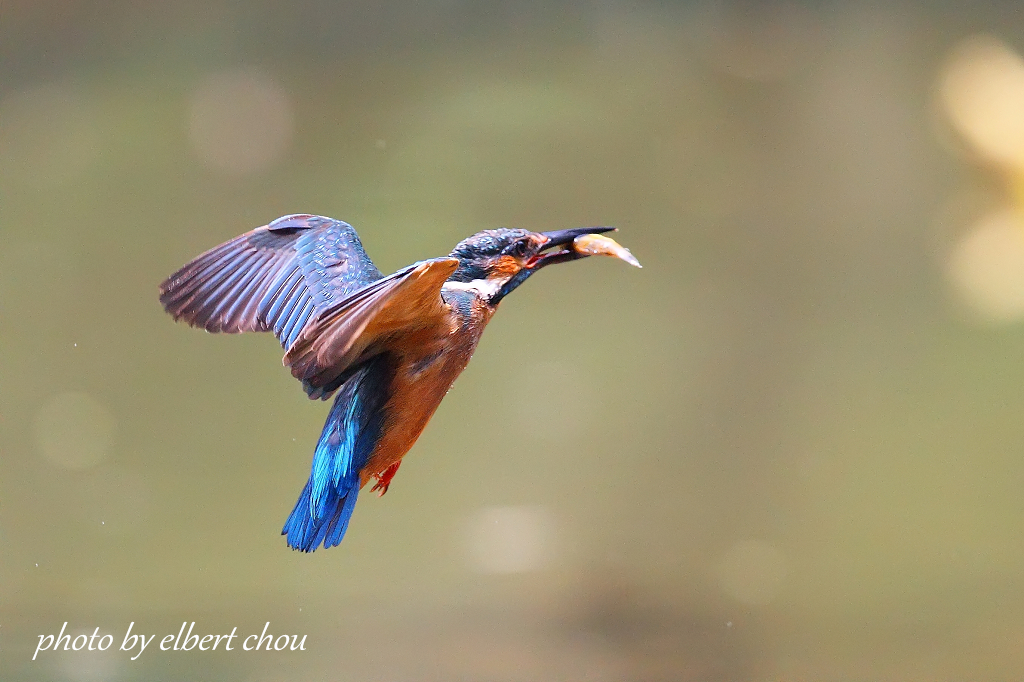This photograph captures a vibrant hummingbird in mid-flight, its wings fully spread. The bird's underbelly and wing undersides are a striking orange, while the tops of its wings display a mix of turquoise and royal blue feathers, with the head adorned in navy blue and touches of orange along the sides. The beak is black, open, and clutching a small fish. The hummingbird's eye is a dark, deep shade, either black or brown. The background is a gradient blend of greens, lightening towards the center with diffused yellow spots indicating sunlight. The upper and lower portions of the backdrop shift to darker greens, with two bright yellow splotches on the top left and additional blurred light patches throughout. In the bottom right corner, italicized white text reads "photo by Albert Chu." The overall scene is infused with natural light, complementing the bird’s vivid colors.